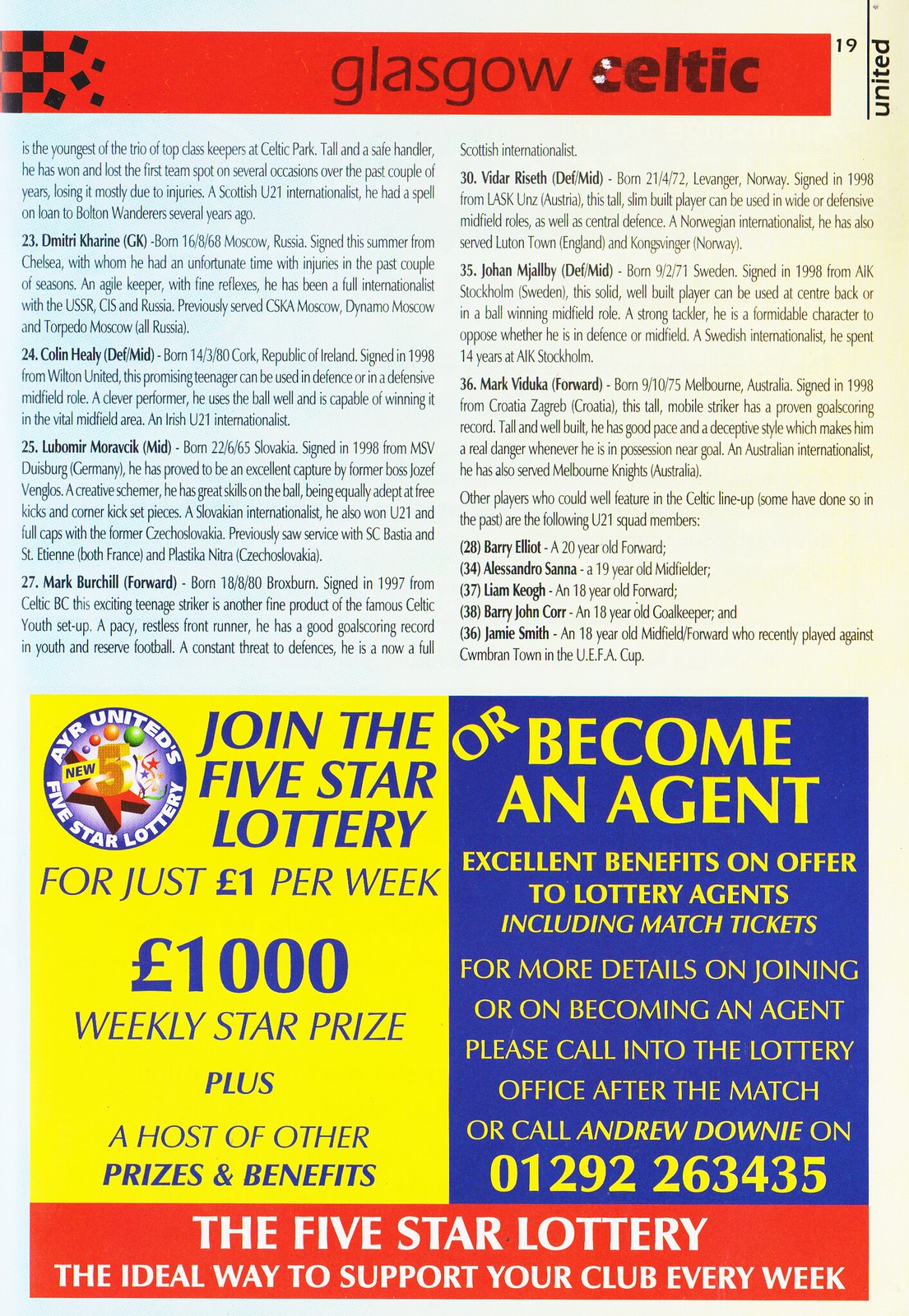The image is of an advertisement or magazine page centered around Glasgow Celtic. Dominating the top of the image is a red rectangle featuring the text "Glasgow Celtic" in black, accompanied by black dots shaped like a soccer ball. Below this, the page is split into two main columns filled with text in small black font, detailing player biographies and their career highlights, including players from various national backgrounds such as Scottish, Russian, Irish, Slovakian, and Norwegian internationals.

The lower section of the image is divided into two parts:
- On the right, there's a dark blue sign with yellow text, inviting readers to "become an agent" with "excellent benefits on offer to lottery agents including match tickets." It provides contact information: "Andrew Downey at 01292 263 435."
- On the left, a section with a yellow background and dark blue text promotes the "five-star lottery," stating, "Join the five-star lottery for just one pound per week and a 1,000-pound weekly star prize plus a host of other prizes and benefits."

At the very bottom of the image, a red strip with white letters reads, "The five-star lottery: The ideal way to support your club every week."